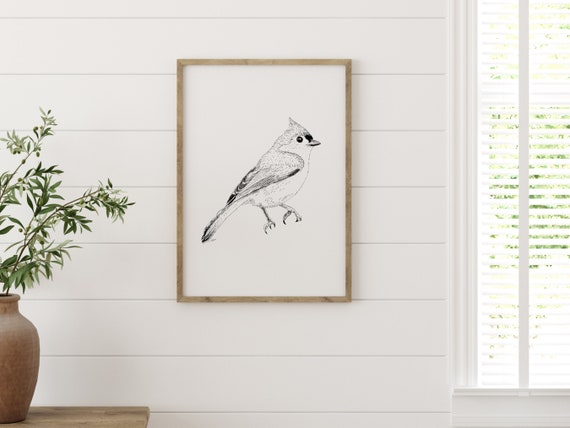The image captures a serene and clean living room with white brick walls. The focal point is a delicately hand-drawn black and white portrait of a cardinal, framed by a thin, light wood border, which accentuates the articulate details of the bird's face, feathers, and feet. This framed drawing is centrally mounted on the wall, enhancing the room's neutral tones. To the bottom left, a green plant in a red vase rests atop a blurry wooden table, adding a subtle touch of color to the minimalist decor. On the far right, sunlight filters through partially open vinyl blinds, casting a bright yet soft light, revealing hints of green foliage outside. The overall composition exudes a sense of calm and meticulous simplicity.